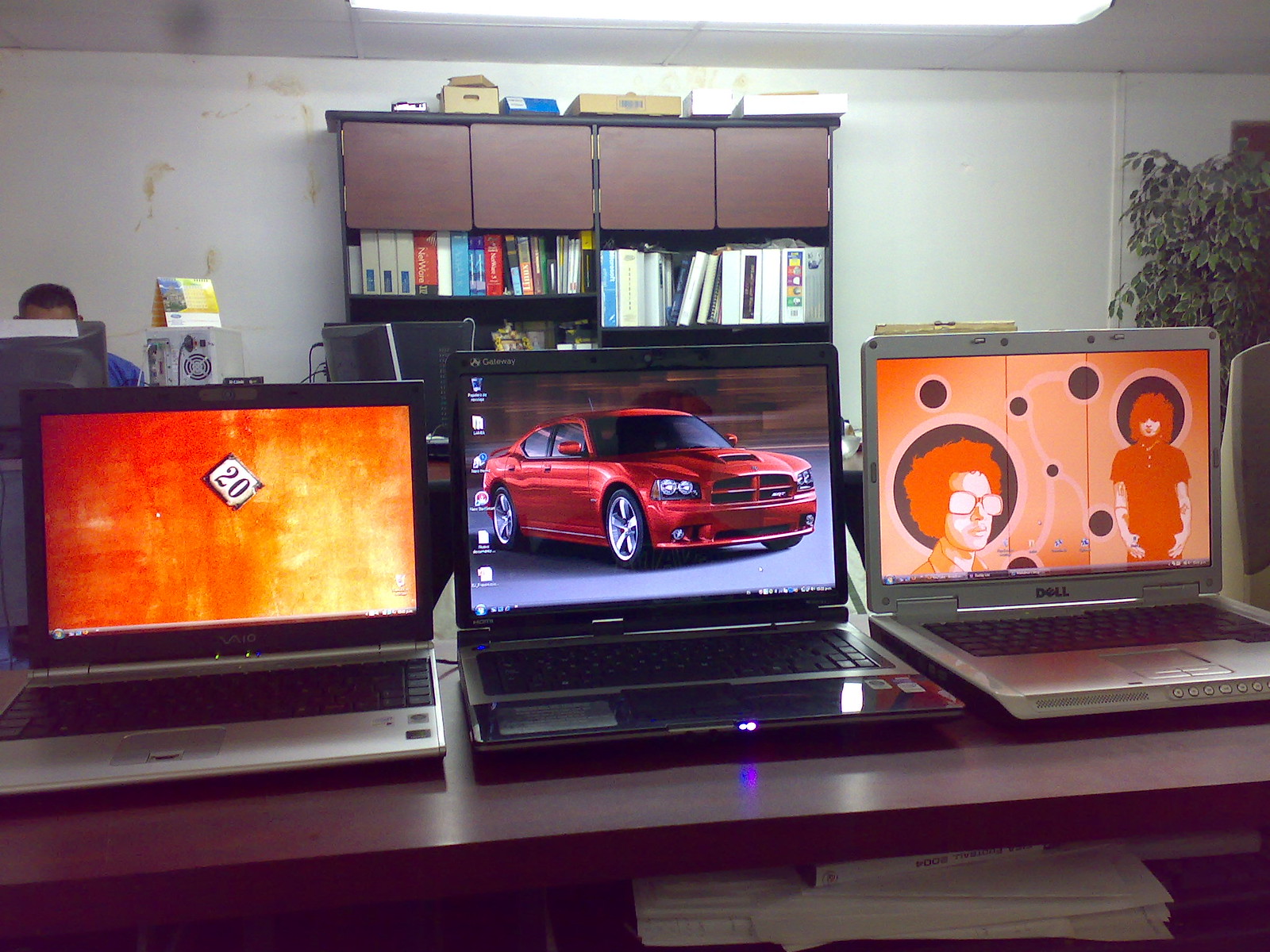The image shows a classroom-like office setting with three laptops positioned on a walnut desk in the foreground. The laptops, which have slightly outdated designs, display distinct screensavers: the left one features an angled number "20" on an orange and gold background, the middle one showcases a bright red sports car against a grey and brown backdrop, and the right one displays cartoon-like characters amid an orange bubble-like design. Behind the desk is a large shelving unit filled with binders, books, and potentially old VCR tapes. On the left side of the image, an African-American man in a blue shirt is focused on a desktop computer with numerous cables connected to a tower beside him. The workspace is brightly lit by a large overhead light, and a big plant adds a touch of greenery to the scene.